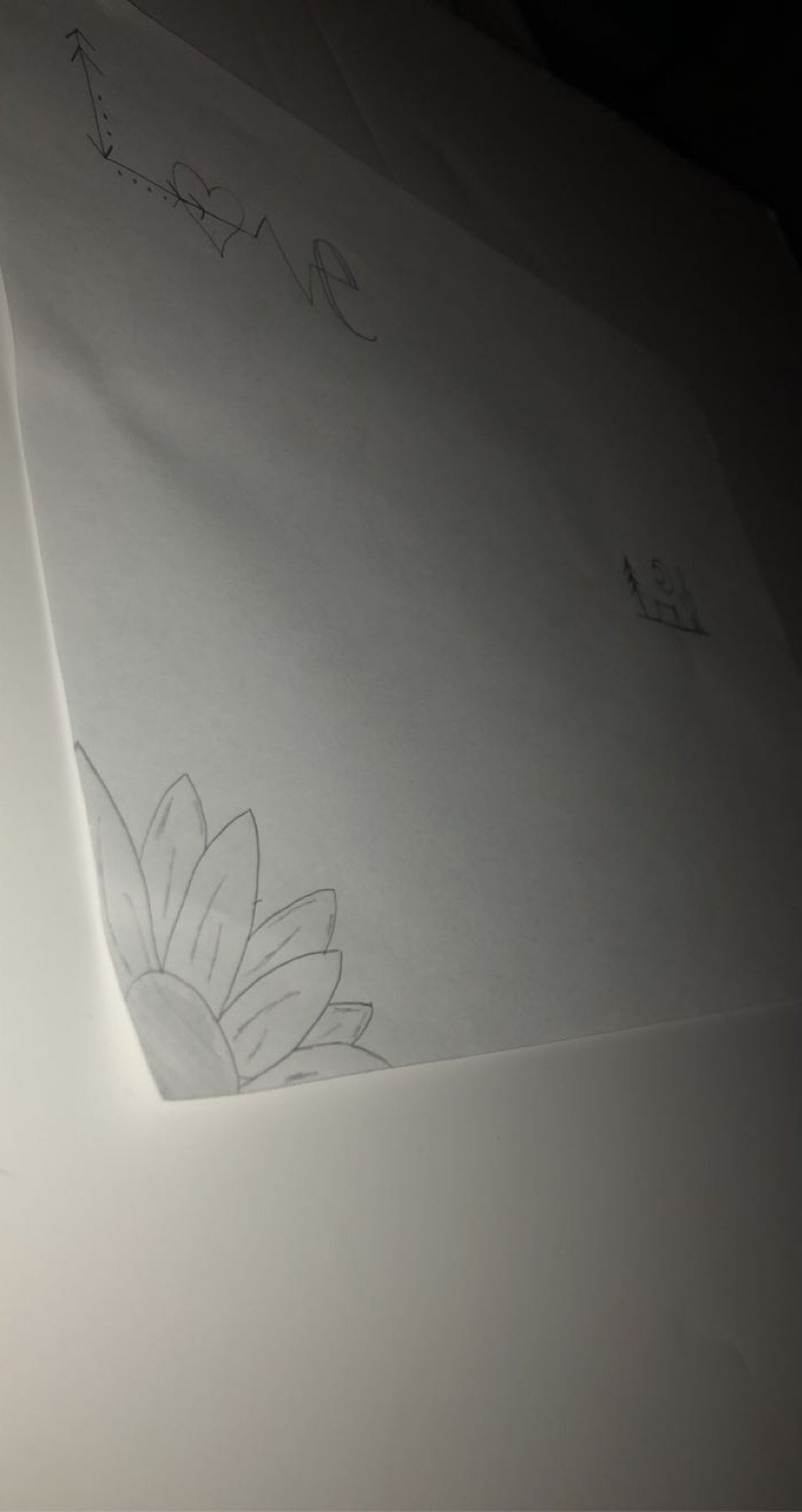On top of a pristine white countertop lies a piece of paper adorned with various artistic elements. In the top left corner, the word "LOVE" is prominently featured, with the "O" creatively replaced by a heart shape. This gives the word a warm and affectionate feel. Adjacent to the word "LOVE" are several small images that add to the paper's charm. The bottom left corner is decorated with a detailed illustration of a flower, consisting of a heart-shaped center and five symmetrical petals, radiating outward. Finally, the top right corner of the paper is embellished with a simple, yet elegant heart. The overall design exudes a sense of love and care, thoughtfully illustrated on the paper.